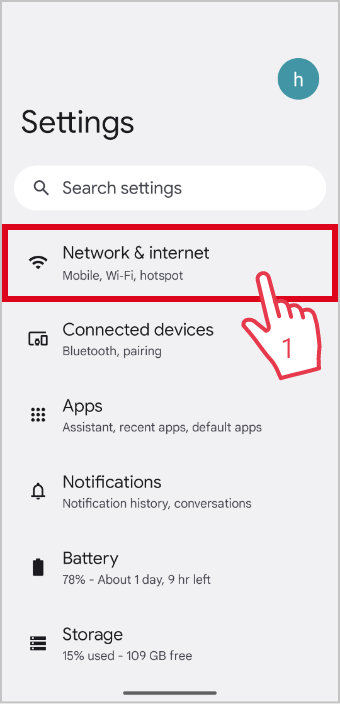The image showcases a device settings screen with multiple sections. In the top right corner, there is a light purple box containing a blue circle with an "H" inside it, and the word "Settings" displayed to the left. Immediately beneath this is a search bar. 

Prominently, there is a red box highlighting the "Network and internet" section, which includes options like "Mobile" and "Wi-Fi hotspot." An illustrated red hand with its index finger pointing upwards is placed within this red box, and it features a red number seven on the back of the hand.

Below the highlighted section, additional categories are listed, including "Connected devices" for managing Bluetooth and pairing options. Further down are "Apps," subdivided into Assistant, recent apps, and default apps. Following this, "Notifications" covers notification history and conversations. 

Further details in the image include battery status, indicating 78% remaining with an estimated time of about one day and nine hours left, and storage information showing 15% used and 109GB free. The bottom of the image is outlined with a black line, framing the lower portion of the screen.